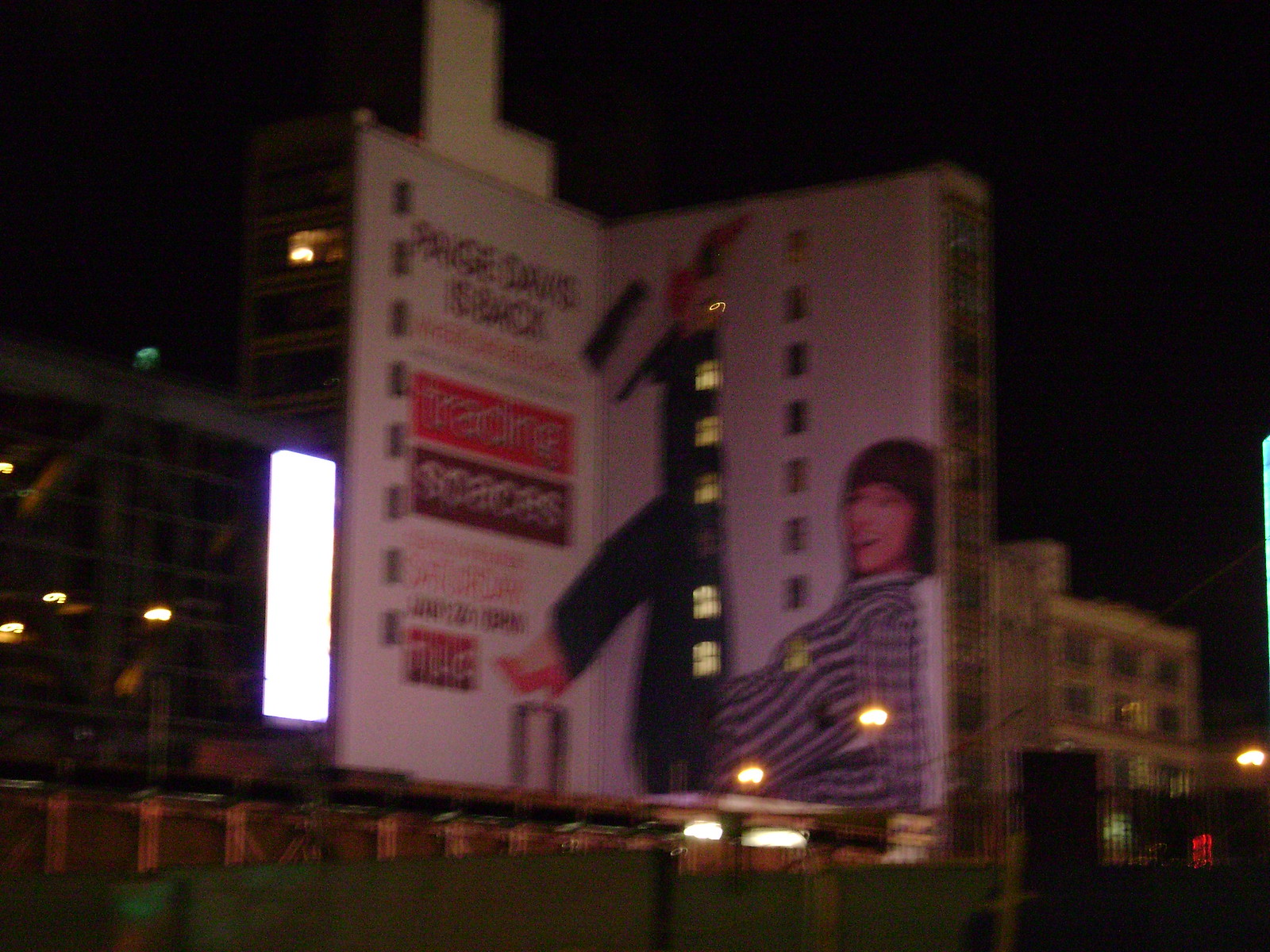A nostalgic, blurry photograph captures an illuminated billboard from the 1970s at nighttime. The central figure on the billboard is a woman, depicted in a stylized drawing typical of the era. She has shortish hair and appears to be Caucasian. She is casually reclining on her back with her hands supporting her, legs playfully raised, adorned in striking red high heels, black jeans, and a long-sleeved striped shirt. The billboard announces "Paige Davis is back" and references snacks, though specific details are obscured by the photo's poor quality and blur. The billboard itself seems to be situated near a transportation hub, its lights cutting through the darkness, lending a sense of vibrant urban life.